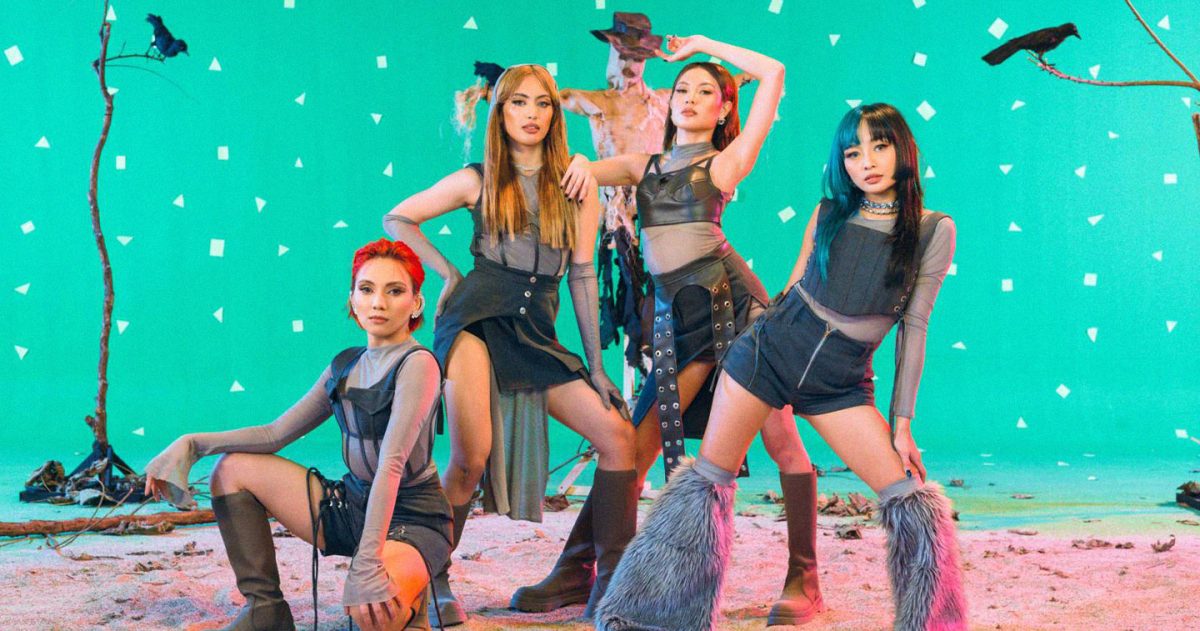This is an indoor, colored photograph depicting a possible music video or photo shoot featuring a young Asian girl band, likely of Filipino origin. The four members, aged around 18 to 19, are dressed in coordinated black and gray outfits, including crop tops, shorts, skirts, leather adornments, and knee-high boots, exhibiting an edgy, artistic style. 

The woman on the far left, who has bright red hair, is kneeling down, wearing gray shorts with leather accents, and brown-toed boots. Beside her, two of the women are standing close to each other; one has long red hair, a gray skirt with three snaps, brown boots, and a gray-striped top with chiffon panels. She leans on a bandmate with shoulder-length black hair, in a sleeveless black crop top and leather skirt, wearing black boots. The fourth woman on the right has long black hair parted in the middle, dressed in gray shorts, a matching gray top with sheer chiffon sleeves, and furry gray boots.

The background, an illuminated green-teal screen with white squares and triangles, suggests an artificial setting. The ground appears sandy, colored pinkish due to yellow and pink lighting. Two stark trees, likely artificial, stand on either side, each adorned with a crow. Centered behind the group is a somewhat ominous scarecrow, taller than the women, wearing a worn brown hat and holding a gun. The entire scene conveys a visually striking, surreal atmosphere.